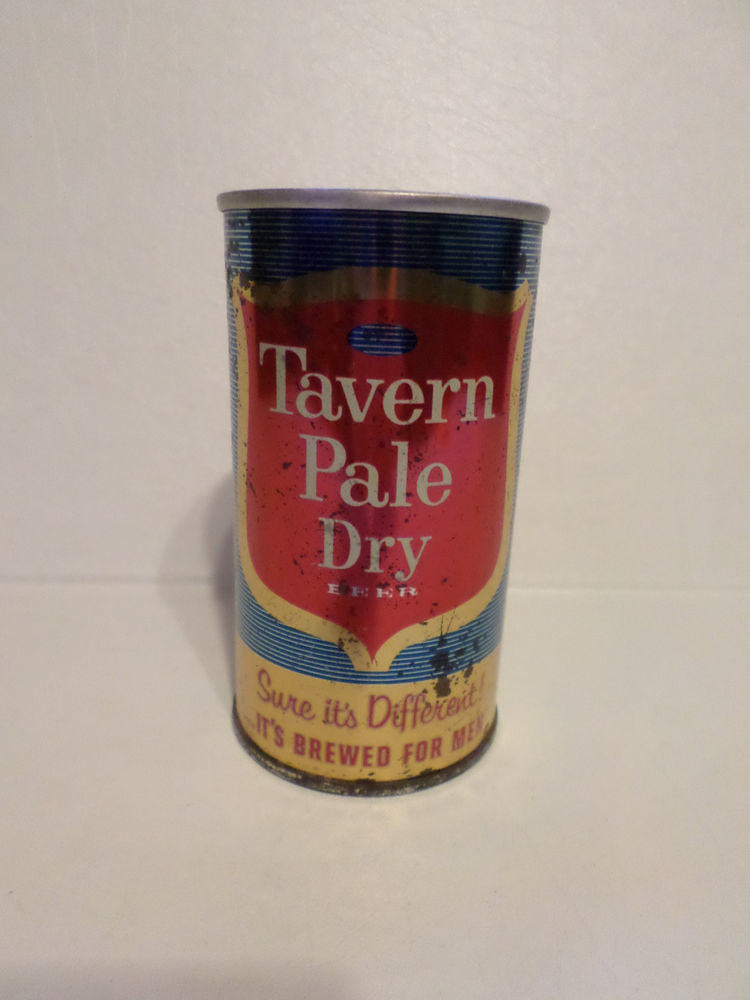This image features a close-up, portrait-oriented photograph of a tall, thin, and very old beer can resting on a white surface against a white background. The can, which looks beat-up and slightly rusted, particularly around the bottom rim, has a distinctive vintage design. The label appears to be directly printed onto the tin, featuring a primarily blue color scheme with various graphic elements. 

Central to the design is a gold-outlined shield with a red interior, housing white text that reads "Tavern Pale Dry Beer." Beneath this shield is a yellow ribbon banner with red script stating, "Sure it's different, it's brewed for men." The tagline uses thin lowercase letters for the first sentence, while "it's brewed for men" is rendered in all-uppercase thick red lettering, emphasizing its bold statement. The image is striking not only for the can's retro aesthetic and noticeable wear but also for the intriguing and somewhat archaic branding.